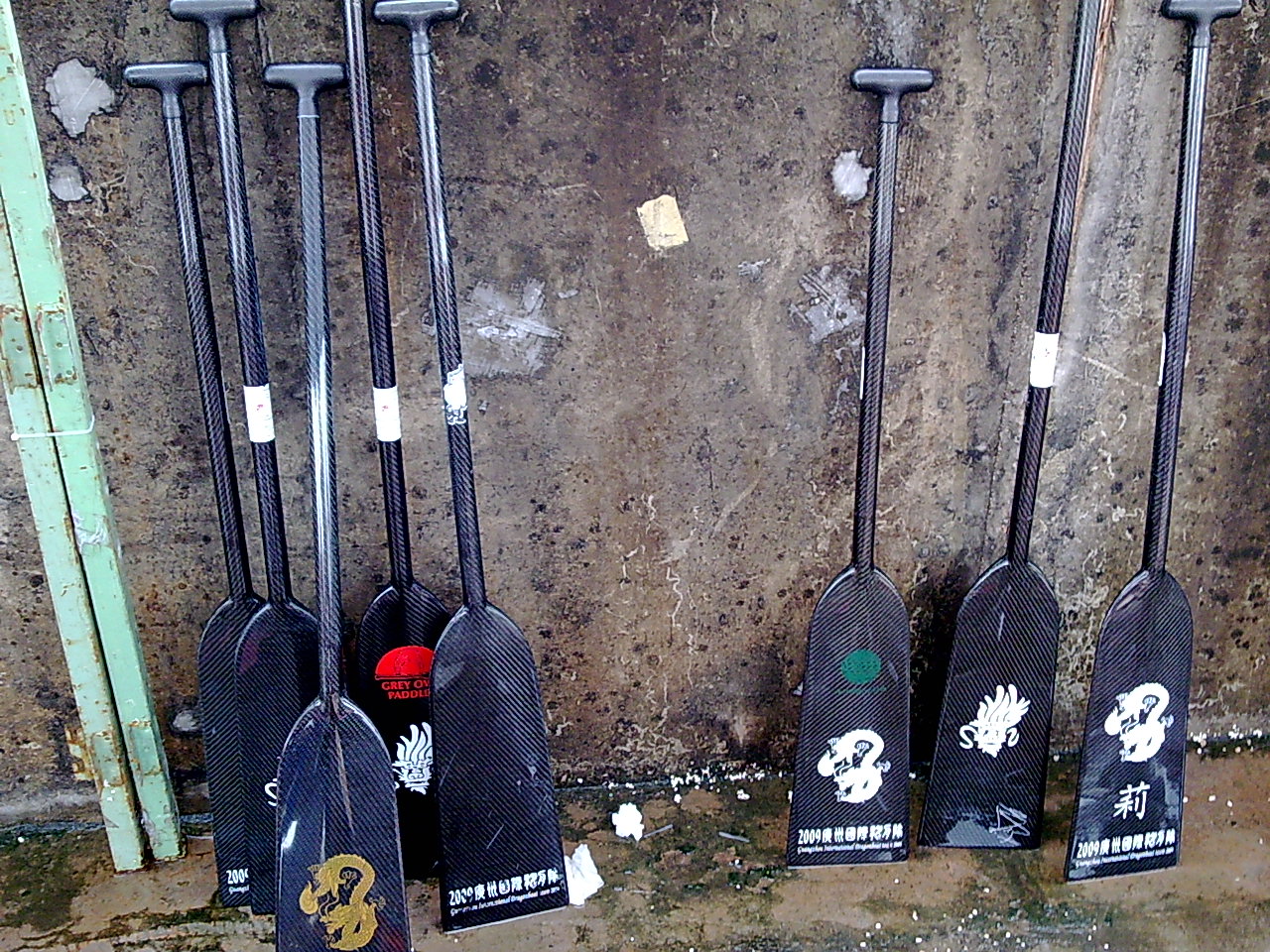The image features an old, dirty cement wall with a speckled look, accentuated by black patches of dirt and age. On the floor, which appears to be concrete with hints of green algae, stand two tall green poles on the left side, possibly parts of a door. Leaning against this wall are eight distinctive oars that vary slightly in height, with five on the left and three on the right, separated by a noticeable gap. These oars, made of either plastic or metal, are approximately three feet tall and adorned with various decorations and symbols. Among the designs are white skull logos, a face with big hair in white, and a gold snake. Some oars feature red elements and characters, possibly in Asian script, with intricate prints. The oars collectively create a striking visual against the aged, grimy backdrop of the cement wall.